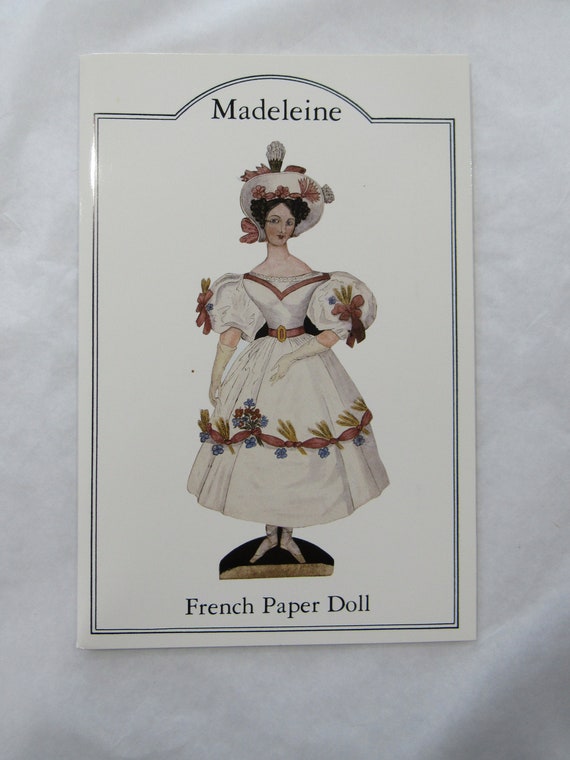The image is a poster with a grayish-white marble textured background that gives it a distinctive antique feel. The poster itself has a white background bordered by two gray, double-lined borders that create a neat rectangular frame. At the top center, within a semi-circular curve in the border, the name "Madeleine" is prominently displayed in silver or dark black letters. Below, the text "French Paper Doll" is equally noticeable at the bottom.

The central illustration is of a detailed and elegant paper doll. The doll is depicted as a sophisticated woman with brown hair elegantly styled up. She wears an elaborate white hat adorned with flowers, leaves, and a poofy white decoration on top, complementing her ensemble. 

Her dress is a striking white garment with a V-neckline and voluminous, puffy sleeves that reach just above the elbow. The dress features intricate vine-like designs with flowers and leaves, adding a touch of botanical charm. Around her waist, she sports a gold belt, and she's adorned with cream-colored gloves that accentuate her refined appearance. Her entire outfit, including the decorative elements on her sleeves and her matching slippers, speaks of classic elegance. The doll stands poised on a small platform, making her appear even more graceful within the poster.